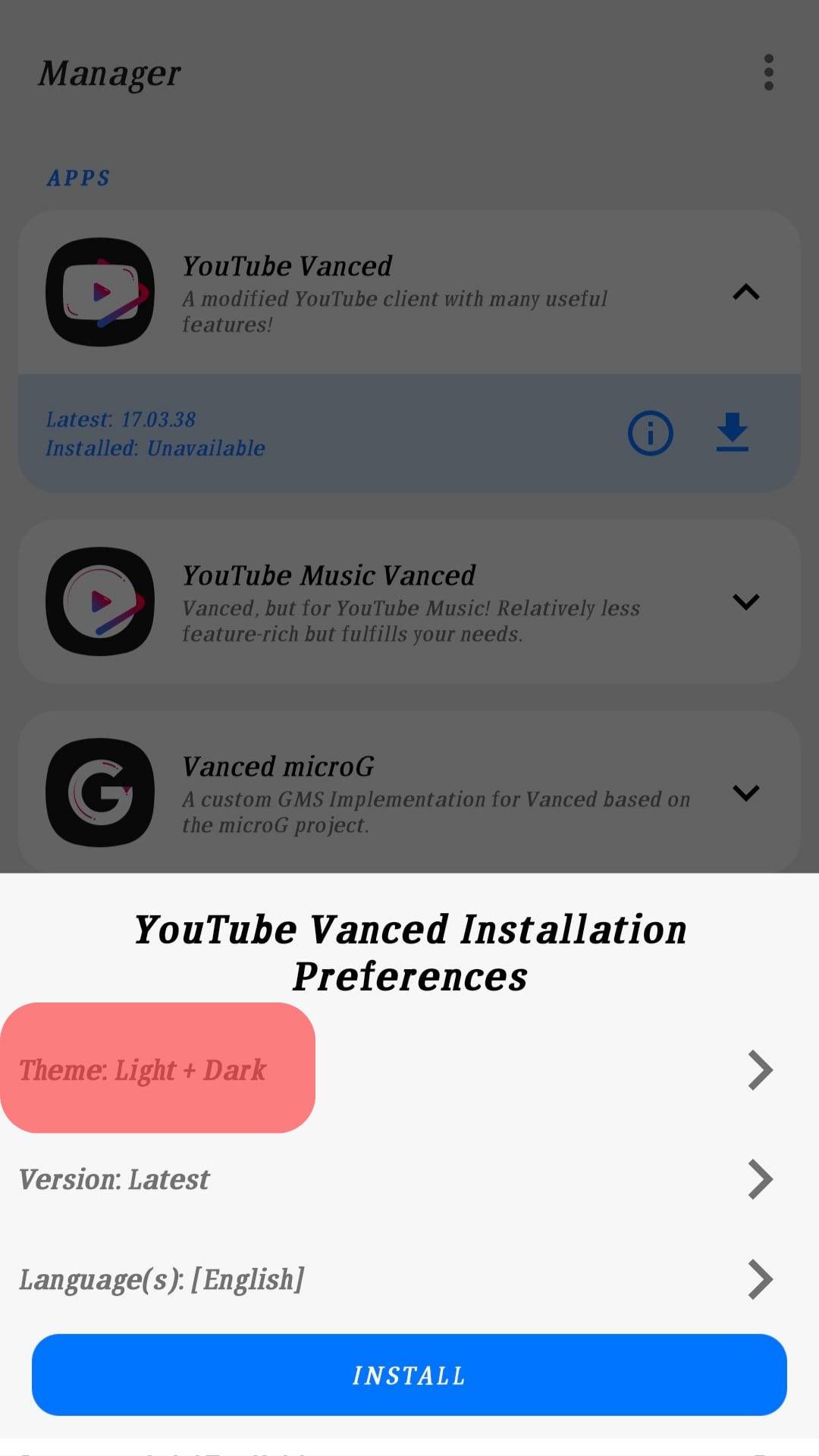**Detailed Caption:**

The image depicts a vertical screenshot of a mobile app interface, presumably designed for managing other applications. At the top left corner of the screen, the label "Manager" is visible, indicating the section of the app. To its immediate right, there's a vertical ellipsis (three stacked dots), serving as the Settings button.

Below this header, the screen lists a series of applications. The first app listed is "YouTube Vanced," described as a modified YouTube client with many useful features. The latest version available is 17.03.38, although the status indicates it is currently "unavailable" for installation. Adjacent to this status is a small information icon (a lowercase "i" encircled in blue) and a blue "Download" button, which appears to be currently selected.

Following this, the next app listed is "YouTube Music Vanced," which is a version of Vanced tailored for YouTube Music. While it offers relatively fewer features compared to YouTube Vanced, it still meets essential user needs. This entry includes a drop-down option for further configurations.

The final app listed in this section is "Vanced MicroG," described as a custom GMS implementation for Vanced based on the MicroG project, also featuring a drop-down option for additional settings.

The lower part of the screen, distinguished by a brighter white background, is dedicated to "YouTube Vanced Installation Preferences." Here, the user can select the theme, currently set to "Light Vast Dark" with a red oblong selection button. Below this, the version is marked as the "Latest," the language is set to "English," and a blue "Install" button awaits user interaction.